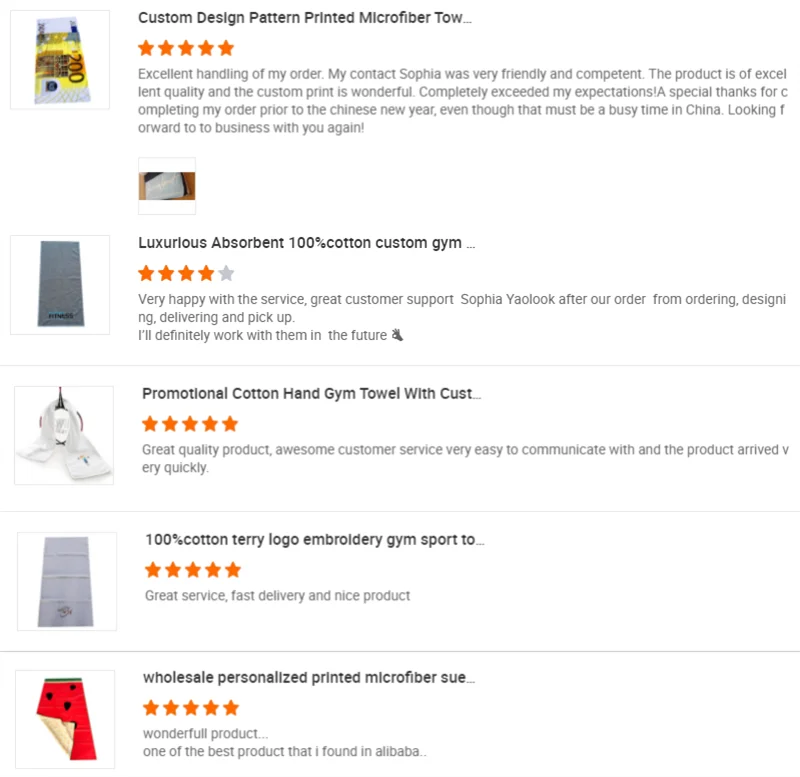**Detailed Customer Reviews of Custom Printed Microfiber Towels and Cotton Gym Towels**

**Review Summary:**

1. **Custom Design Pattern Printed Microfiber Towel** - **Five Stars**
   - **Review**: Excellent handling of my order. My contact, Sophia, was very friendly and competent. The product is of excellent quality, and the custom print is wonderful, completely exceeding my expectations. Special thanks for completing my order prior to the Chinese New Year, despite the busy time. Looking forward to doing business again.
   - **Images**: Two small images of the product, likely showcasing the custom design, though details are hard to see.

2. **Luxurious, Absorbent 100% Cotton Custom Gym Towel** - **Four Stars**
   - **Review**: Very happy with the service and great customer support. Sophia Yao looked after our order from beginning to end. I'll definitely work with them again in the future.
   - **Images**: To the left, an image of a gray towel.

3. **Promotional Cotton Hand Gym Towel with Custom Design** - **Five Stars**
   - **Review**: Great quality product, awesome customer service, very easy to communicate with, and the product arrived very quickly.
   - **Images**: The image seems to be of a white towel, though it’s a bit unclear.

4. **100% Cotton Terry Logo Embroidery Gym Sport Towel** - **Five Stars**
   - **Review**: Great service, fast delivery, and a nice product.
   - **Images**: Another gray towel, this one a lighter shade.

5. **Wholesale Personalized Printed Microfiber Towel** - **Five Stars**
   - **Review**: Wonderful product, one of the best products that I have found on Alibaba.
   - **Images**: Towel with a watermelon design, the lower left corner of the towel is flipped up.

**Note**: Most images accompanying reviews are small, making detailed inspection difficult. However, all feedback highlights excellent service and high-quality products.